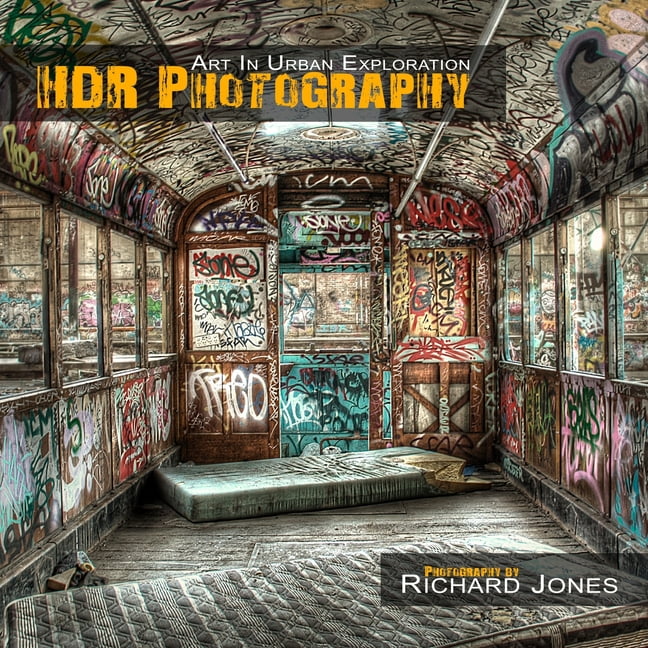The image appears to be an advertisement for a photography studio or art gallery exhibit, prominently displaying urban exploration and HDR photography. The text includes "Art and Urban Exploration" in white at the top, "HDR Photography" in a yellowish-orange, and "Photography By Richard Jones" in white at the bottom right, set against a matching yellowish-orange background. The focal point of the photograph is the interior of an old, abandoned train car, which is fully graffitied in an array of vibrant colors such as pinks, blues, greens, reds, and every imaginable hue. The train car's floor is littered with a couple of worn-out mattresses, adding to the scene's dilapidated and gritty atmosphere. The walls and surfaces are extensively tagged with various names and street art, reflecting the raw, urban essence captured by Richard Jones in this immersive HDR photograph.